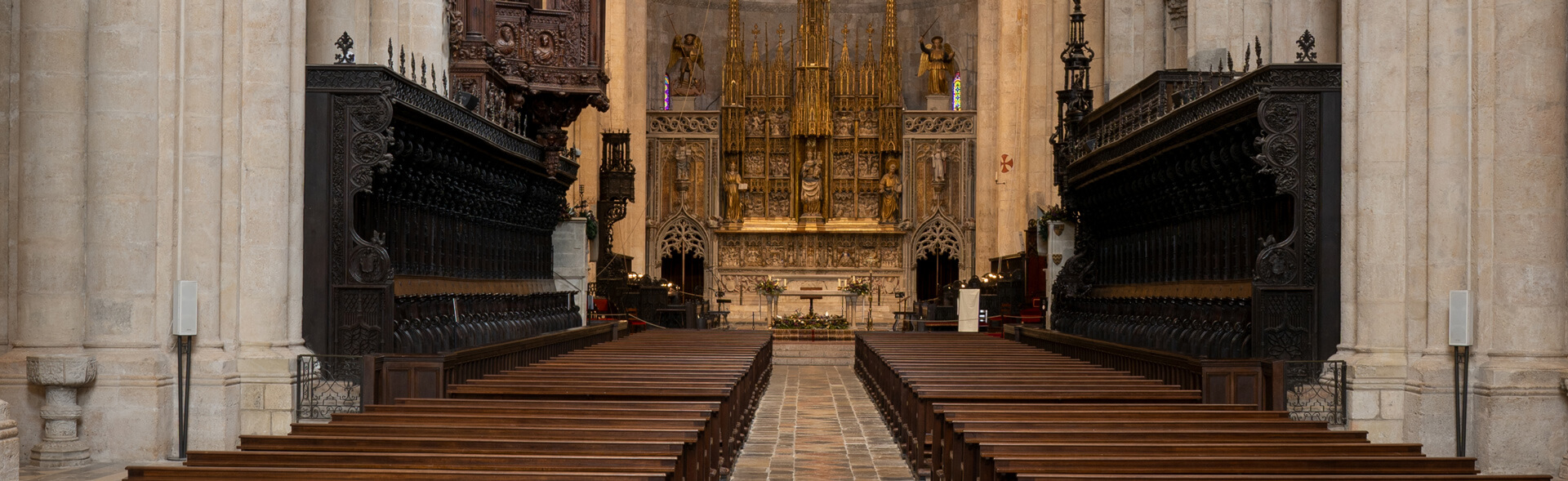The photograph depicts the interior of a grand, old Catholic church, likely a cathedral, taken from the viewpoint of someone standing near the entrance and looking down the stone-paved aisle. The cathedral's architectural details are magnificent and intricate. On either side of the central aisle are rows of wooden benches. These benches are partially enclosed within structures resembling small houses with roofs.

The aisle itself leads to a splendid sanctuary framed by two white marble pillars supporting grand arches. Nestled within this sanctuary are three sculptures—potentially depicting religious figures, with the central statue possibly representing Saint Mary holding baby Jesus. Flanking the central statue are figures that could be saints, with additional statues of angels placed atop the pillars, one notably holding a sword.

The church's interior showcases a blend of golden decor and the white marble of the pillars, contributing to a sense of opulence and reverence. Along the walls, candles arranged in what looks like encased bookshelves add to the sanctified atmosphere. The grandness of the church is further emphasized by the presence of a towering pipe organ and various smaller details designed to invoke awe and spiritual reflection.